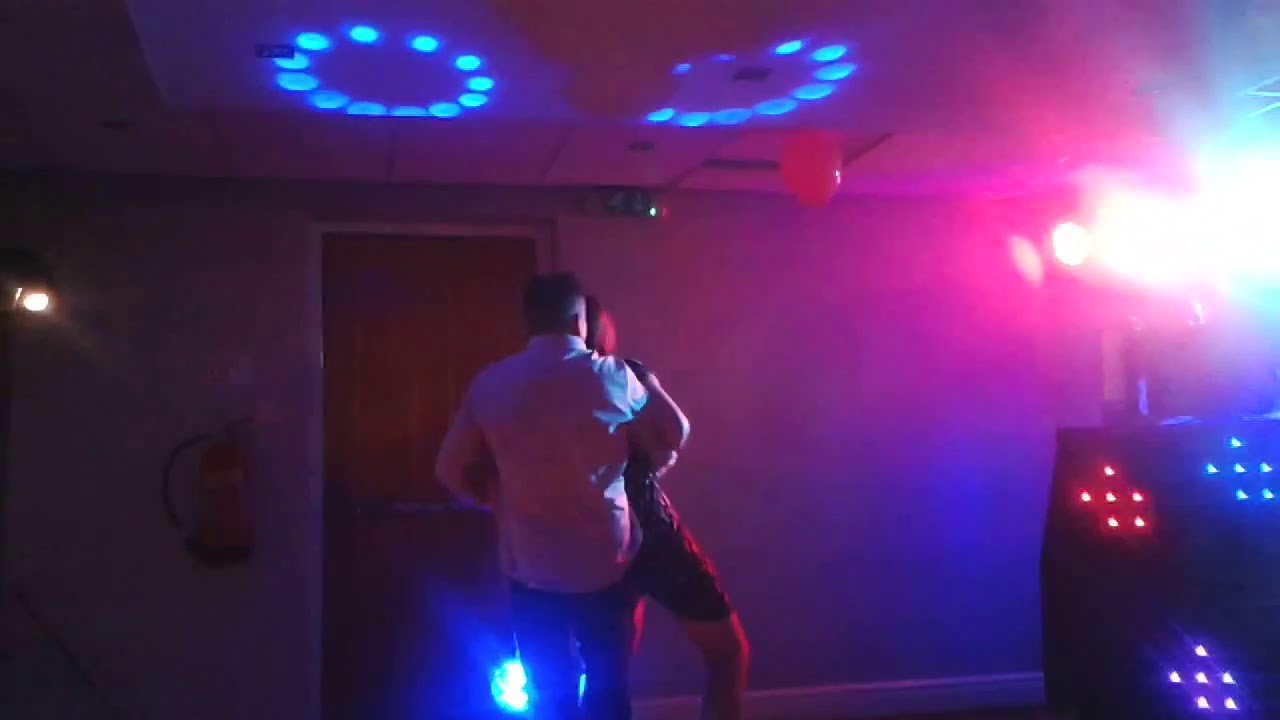The photograph captures a dimly lit, hazy room that resembles a dance floor, possibly in a club or small karaoke bar. The ambient lighting creates an array of colors, predominantly light pink and purple hues, with a blacklight effect adding to the ethereal atmosphere. There are two notable circular arrays of small blue neon lights on the white ceiling, and a red balloon floats near them.

In the center of the image, a man with dark hair, wearing a long button-down collar shirt (which appears off-pink due to the lighting) and black pants, has his back turned to the camera. He seems to be holding a woman, who is partially obscured by him. Only her right leg, which is either in shorts, a skirt, or a black dress, is visible, along with her head and red-tinged hair, which is likely colored by the lighting.

The background showcases a standard wall, adorned with a brown wooden emergency exit door, and a red fire extinguisher mounted to the left of the door. In the bottom-right corner, there is a black machine with red and blue lights, and above it, a bright light further illuminates the room, providing a bluish-purplish glow that adds to the surreal ambiance.